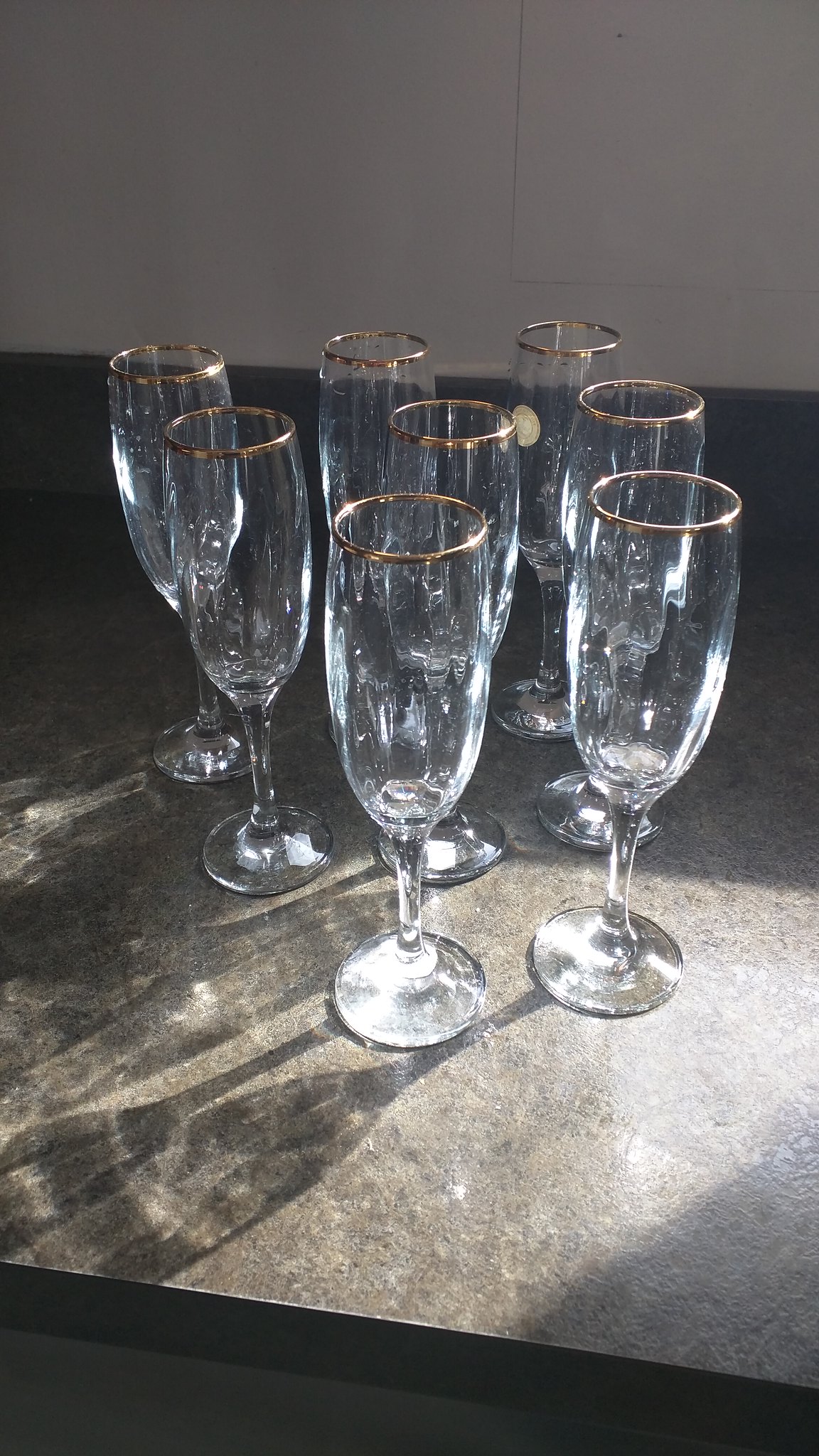The photograph captures a birds-eye view of a granite kitchen countertop, featuring eight identically faceted champagne flutes. The speckled countertop, in hues of gray and brown, provides a striking contrast to the glasses arranged neatly in three columns—two in the first column, and three each in the second and third columns. Each glass, with its slender, elongated body and flat base, glistens under a light source coming from the right, casting subtle shadows downward and to the left. The rim of these champagne flutes is adorned with an elegant bronze-gold finish, adding a touch of sophistication. In the background, a white tiled wall further enhances the clean, bright aesthetic of the image.